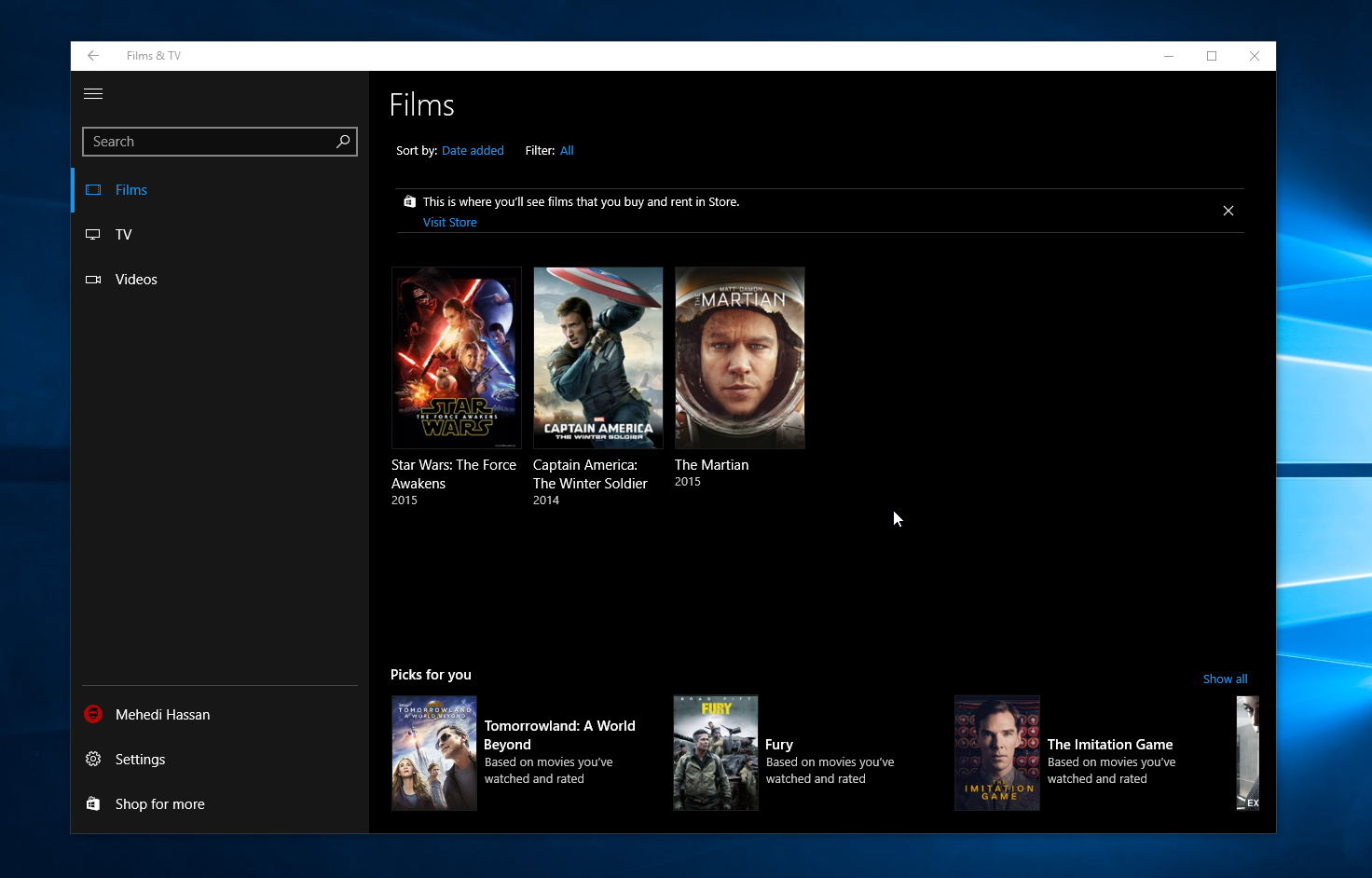The image displays a computer desktop with a blue background wallpaper, acting as a thin border around a prominent black pop-up window. On the left side of the window, there is a vertical navigation column. At the top of this column is a search bar, followed by labeled sections: "Films", "TV", and "Videos". Towards the bottom, the column lists "Michael Hassan", "Settings", and "Shop for More".

The main section of the pop-up window focuses on films. The first row displays three movie thumbnails, each with their respective titles listed below: "Star Wars: The Force Awakens", "Captain America: The Winter Soldier", and "The Martian". 

Below this row, another section labeled "Pics for You" presents three more movie thumbnails. Unlike the first row, the titles for these movies are positioned to the right of their thumbnails. The films in this section are "Tomorrowland: A World Beyond", "Fury", and "The Imitation Game".